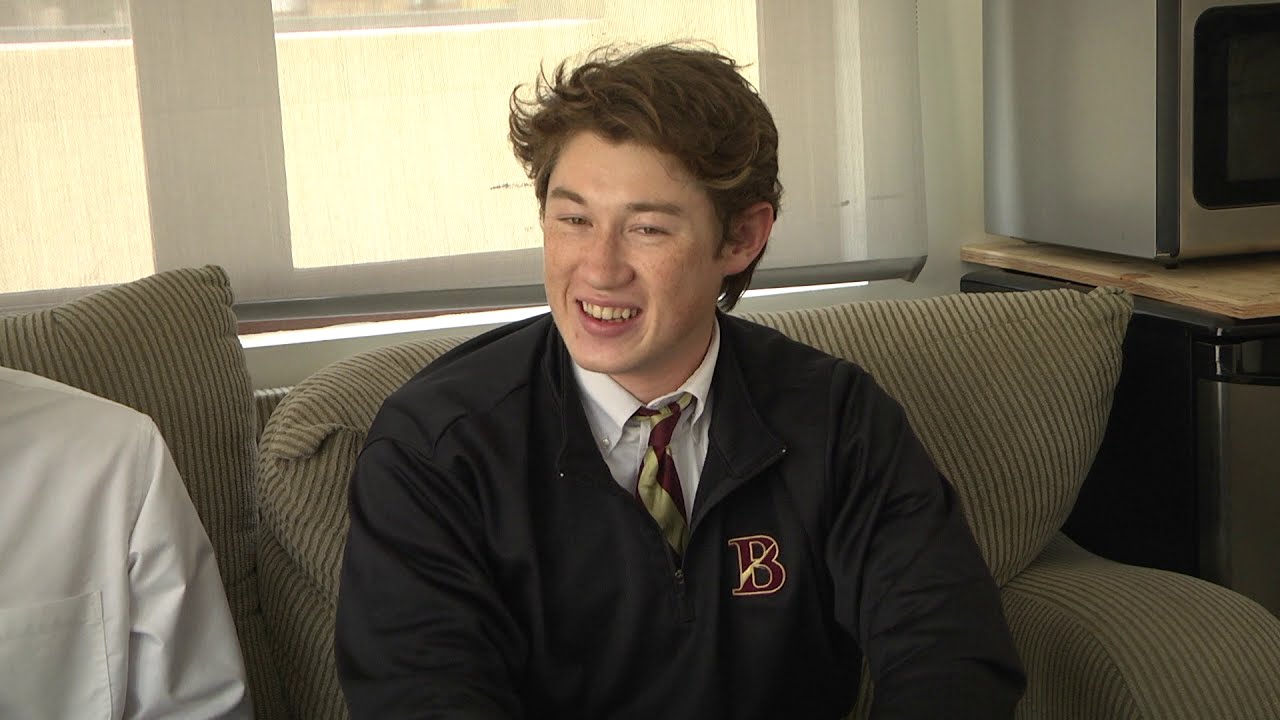In this detailed image, a young man, likely in his late teens, is seated on a tan, cushioned couch with beige and gray stripes. His head is slightly turned to the left as he smiles and looks to the right, revealing his yellow-tinged top teeth. He has unkempt, shaggy brown hair that curls up on the left side and fair skin adorned with freckles.

Dressed in a black zip-up jacket featuring a large capital "B" on the left chest—emblazoned with a distinctive yellow stripe—he also wears a white button-down shirt underneath, complemented by a loosely tied maroon-and-gold striped tie. The couch has large pillows behind him.

In the background, a window with a white frame shows a yellow wall with a white line near the top and a soft yellow light filtering through. To his right, a wooden countertop supports a silver microwave with a tinted window, suggesting a kitchenette area. Additionally, to his left, the shoulder of another person in a white button-down shirt is faintly visible within the frame. This setting gives off a cozy, possibly dormitory-like vibe.